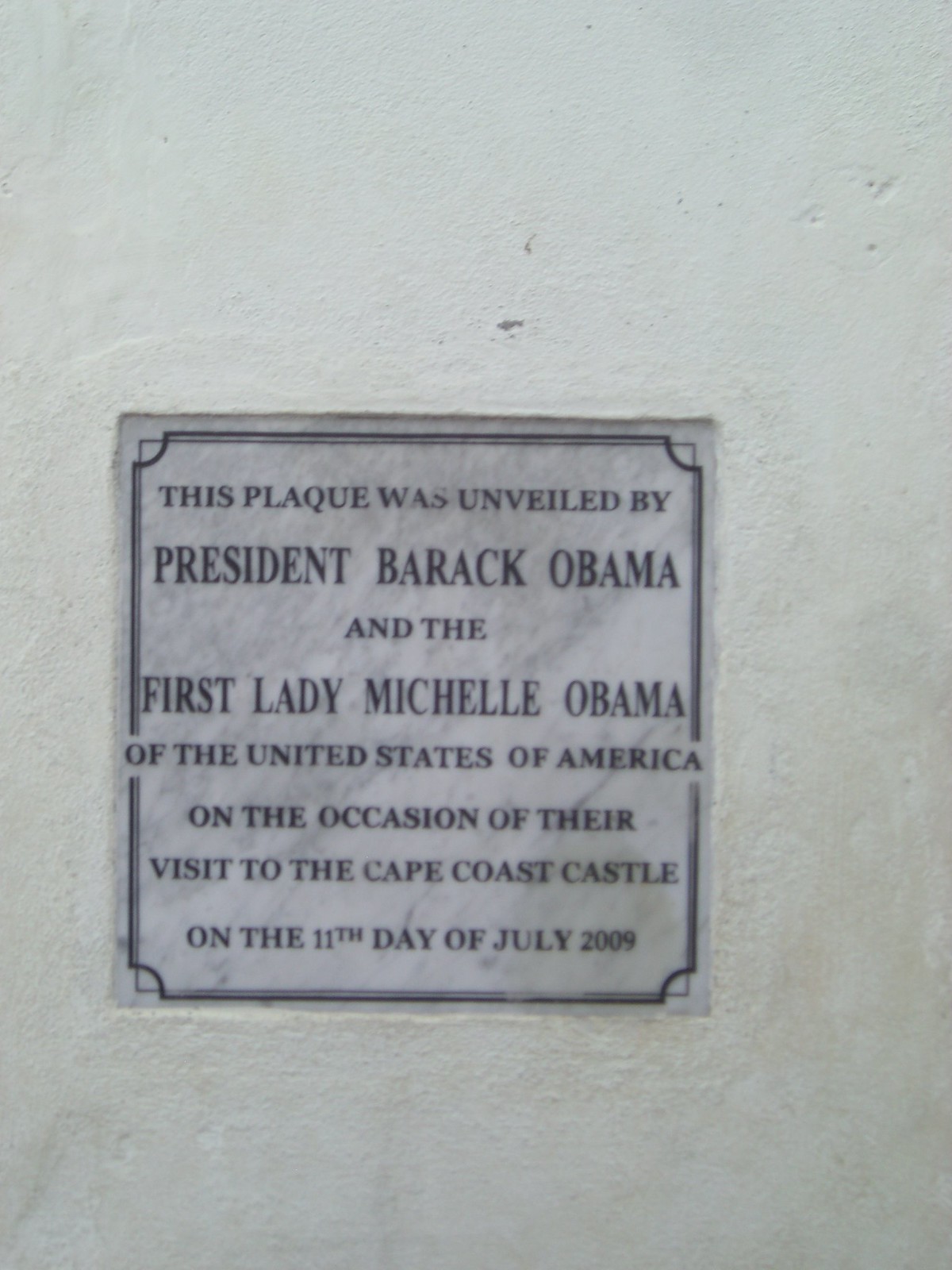The image features a silver plaque embedded into a white stone wall with a slightly marble-like appearance, displaying some chips and discoloration, particularly in the bottom right. The plaque, which appears to be a square slab of whitish-gray marble, is adorned with an ornate black border and another plain black border. The inscription in black text reads, "This plaque was unveiled by President Barack Obama and the First Lady Michelle Obama of the United States of America on the occasion of their visit to the Cape Coast Castle on the 11th day of July 2009." The white painted wall behind the plaque has several marks, dents, and areas where the paint is peeling off or yellowing.